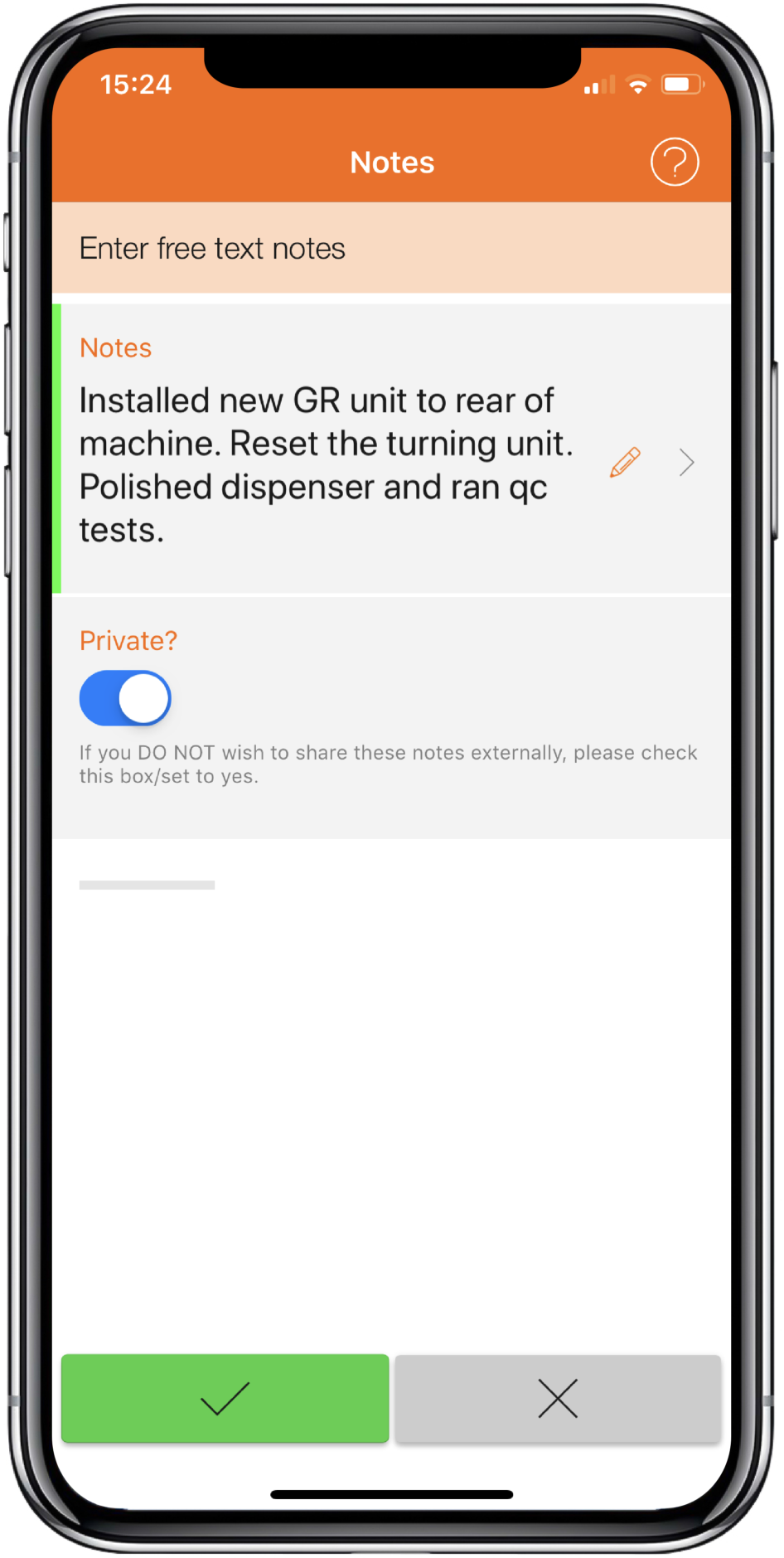The image showcases a mobile device with prominent features clearly visible. The device's power button is located on the right side, while the left side hosts the mute ringer switch at the top, with volume up and down buttons positioned just below it. The screen displays an application interface, featuring an orange bar at the top that contains the word "Notes" centrally. To the right of this bar is a help button, symbolized by a white question mark encased in a circle.

Beneath the orange bar, the interface prompts the user with "Enter free text notes." The text below this header reads: "Notes: Installed new GR unit to rear of machine, reset the turning unit, polished dispenser, and ran QC test." Adjacent to this text on the right, there are icons including a pencil for editing and an arrow pointing to the right, likely indicating navigation or confirmation.

Further down, a gray box with the word "Private" in orange and another question mark icon is displayed. This section includes a toggle button, currently turned on, with a description: "If you do not wish to share these notes externally, please check this box to set to yes." At the very bottom of the screen, there are two options: a green check mark box indicating confirmation, and a gray X box for cancellation or closing the action.